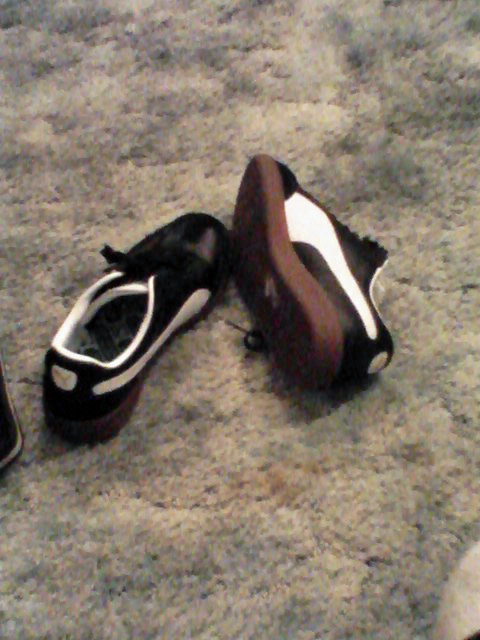This is a detailed photograph of a pair of black Puma sneakers featuring white accents. The sneakers have a distinctive white stripe that curves from the front towards the sole, narrowing as it arches towards the heel in a swoosh-like design. The shoes have black laces, black toe areas, and white linings around the opening and tongues. The back of each shoe displays a patch of white with the Puma logo prominently visible. The soles are a brown color. The left shoe is positioned upright, allowing a clear view inside where the foot would go, while the right shoe is tipped over onto its side, revealing the brown sole and shoelaces underneath the midsection. The shoes are laid out on a plush, grayish-brown shag carpet which has hints of blue and cream throughout, adding to the textured background of the image.